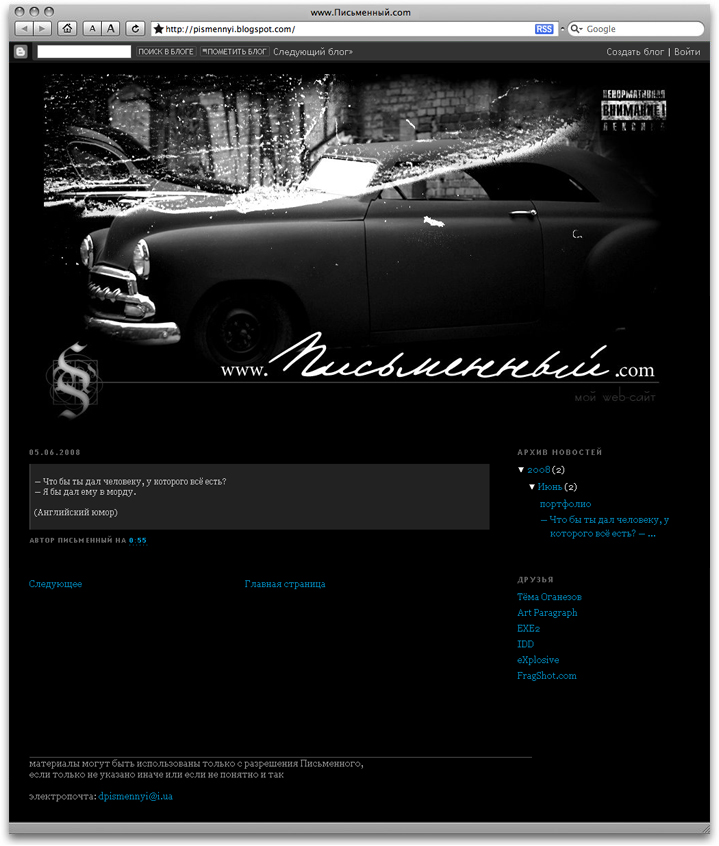The image appears to be a screenshot, likely taken from a Mac or iOS device, showing a webpage with a very dark black background. At the top of the screen, there's a web address, "http://pismenyl.blogspot.com," accompanied by navigation buttons including back, forward, home, reload, and text size adjustment options. The upper right corner displays a Google search bar.

Prominently featured towards the top of the webpage is a nearly silhouetted image of an older-style luxury car, under which is white text displaying "www." However, the following text is mostly illegible, hinting at "www.newcodesomething.com." The rest of the page seems to be filled with text in blue, potentially indicating it is a blog, with a section on the right possibly listing the blog's contents or indices, though this section is difficult to read due to the dark background and varying shades of gray, black, white, blue, and light blue used throughout.